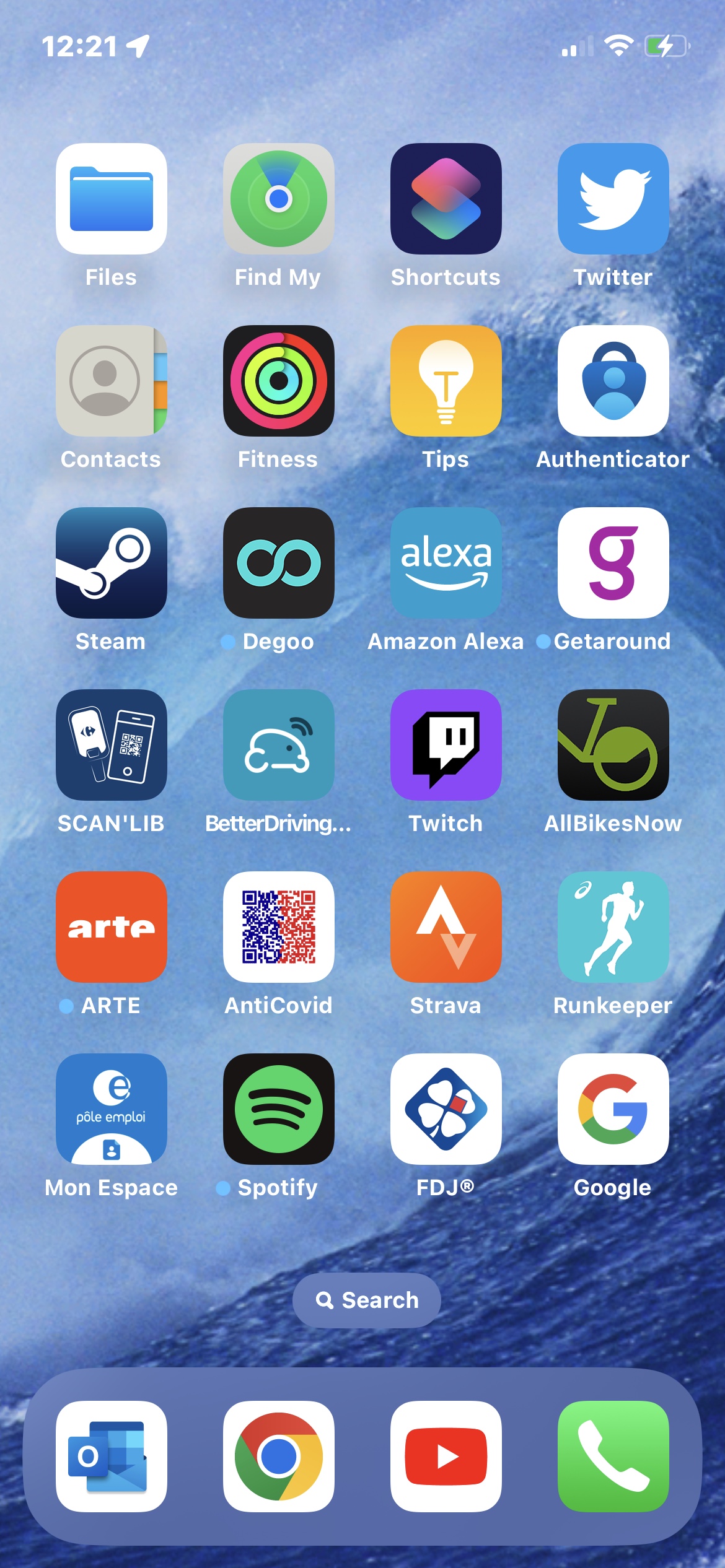Screenshot of a smartphone home screen displaying various app icons neatly arranged in a grid layout. At the very top-left corner, the clock app shows the time as 12:21. In the top-right corner, there is a Wi-Fi signal indicator, a cellular signal bar, and a small battery life icon.

Below these indicators, a grid of apps is visible, organized into four icons per row. Starting from the top-left and moving from left to right, the first row includes the "Files," "Find My," "Shortcuts," and "Twitter" apps. The second row contains "Contacts," "Fitness," "Tips," and "Authenticator." The third row has "Steam," "Daegu," "Alexa," and "Getaround." The fourth row displays "Skin," "Lib," "Better Driving," and "Twitch." Moving to the fifth row, there are the "Old Bikes Now," "Arte," "Anti-COVID," and "Strava" apps. The sixth row holds "Runkeeper," "Bone Escape," "Spotify," and "FDJ." The final row includes the "Google" app.

At the bottom of the screen, there are four icons: an envelope representing the email app, the Google Chrome browser icon, the YouTube app, and the call button.